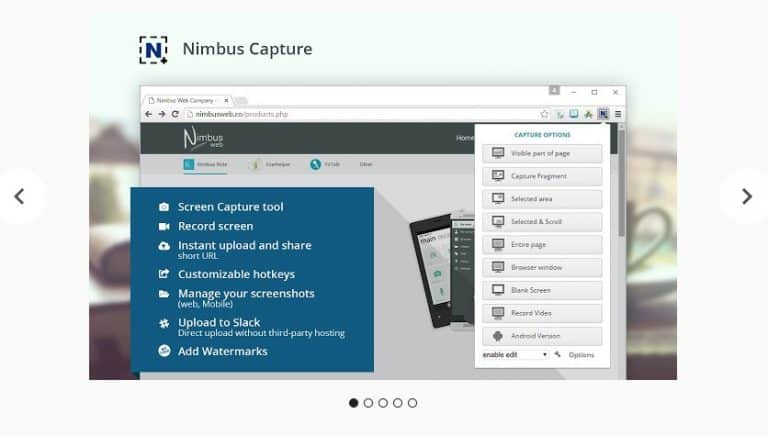A detailed screenshot portrays a user interface of the Nimbus Capture tool. The main feature is a dashed square with a capital 'N' enclosing it, and a plus sign at the lower right corner, possibly indicating an option to add or create something. Below this, a web browser window is open to the Nimbus website, viewed through the familiar interface of Google Chrome. Though the exact URL is unreadable, the page is clearly geared towards Nimbus Web.

On the right side of the browser, a drop-down menu reveals various capture options: a series of icons representing different screen capture functions, including full-screen capture and region-specific capture. The drop-down highlights options such as capturing a visible part of the page, capturing fragments, and selecting a specific area. These options suggest that the software specializes in screen capture capabilities.

Behind this interface, in the background, there's an office photo, which adds a hint of professional context to the scene. On the left side of the screenshot, a text overlay in a blue box lists Nimbus Capture's features. Each feature is paired with an icon: a camera for the screen capture tool, a movie camera for recording screens, and additional icons representing instant upload and sharing with a short URL, customizable hotkeys, management of screenshots for web and mobile, direct uploads to Slack, uploads without third-party hosting, and adding watermarks.

Below this blue overlay, there are images of a smartphone laid out across the web page. Additionally, at the bottom of the screen, five circles indicate a carousel of photos with the leftmost circle currently selected, suggesting navigation through multiple images or pages. This detailed screenshot encapsulates the comprehensive and user-friendly design of the Nimbus Capture interface, highlighting its various functionalities tailored for efficient screen capture, management, and sharing.